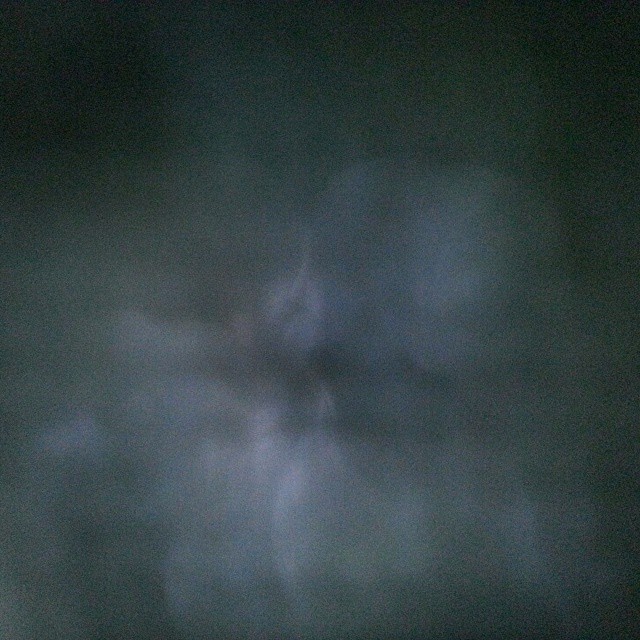The image presents an extremely dark and blurry square photograph with an ambiguous subject. The background exudes a near pitch-black hue with subtle tinges of a dark greenish shade. Positioned centrally, indistinct and faintly white shapes suggest something roundish in form. These shapes, enveloped in heavy blur and poor lighting, vaguely resemble a flower or similar object, but the lack of clarity makes precise identification impossible. Additionally, the image suffers from slight pixelation, further obscuring possible details of the scene.